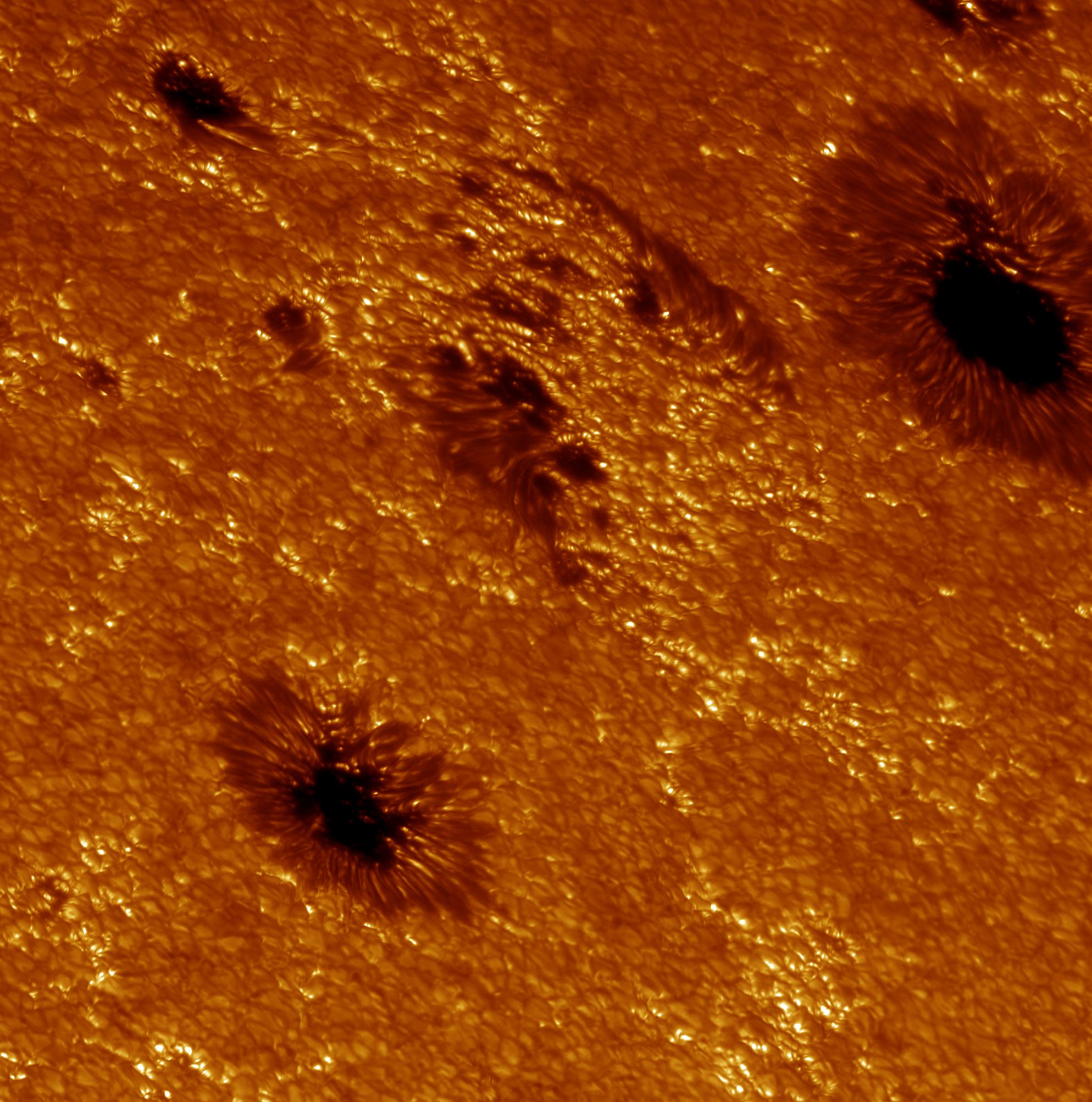The image portrays a highly detailed and textured surface reminiscent of the sun's seething, golden-orange expanse peppered with dark patches. The golden color dominates, interspersed with speckles or flakes that give it a dynamic and almost granular appearance. There are several notable black spots, the most significant of which are located in the top right and bottom left corners, with another smaller but still prominent spot in the top left. These spots strikingly resemble sunspots, with borders that seem to pulse and shift, adding to the impression of movement. Centrally, there are additional smaller spots that haven't yet developed into full black holes, further enhancing the image's complexity and resemblance to a celestial body like the sun or a zoomed-in view of a petri dish under a microscope.